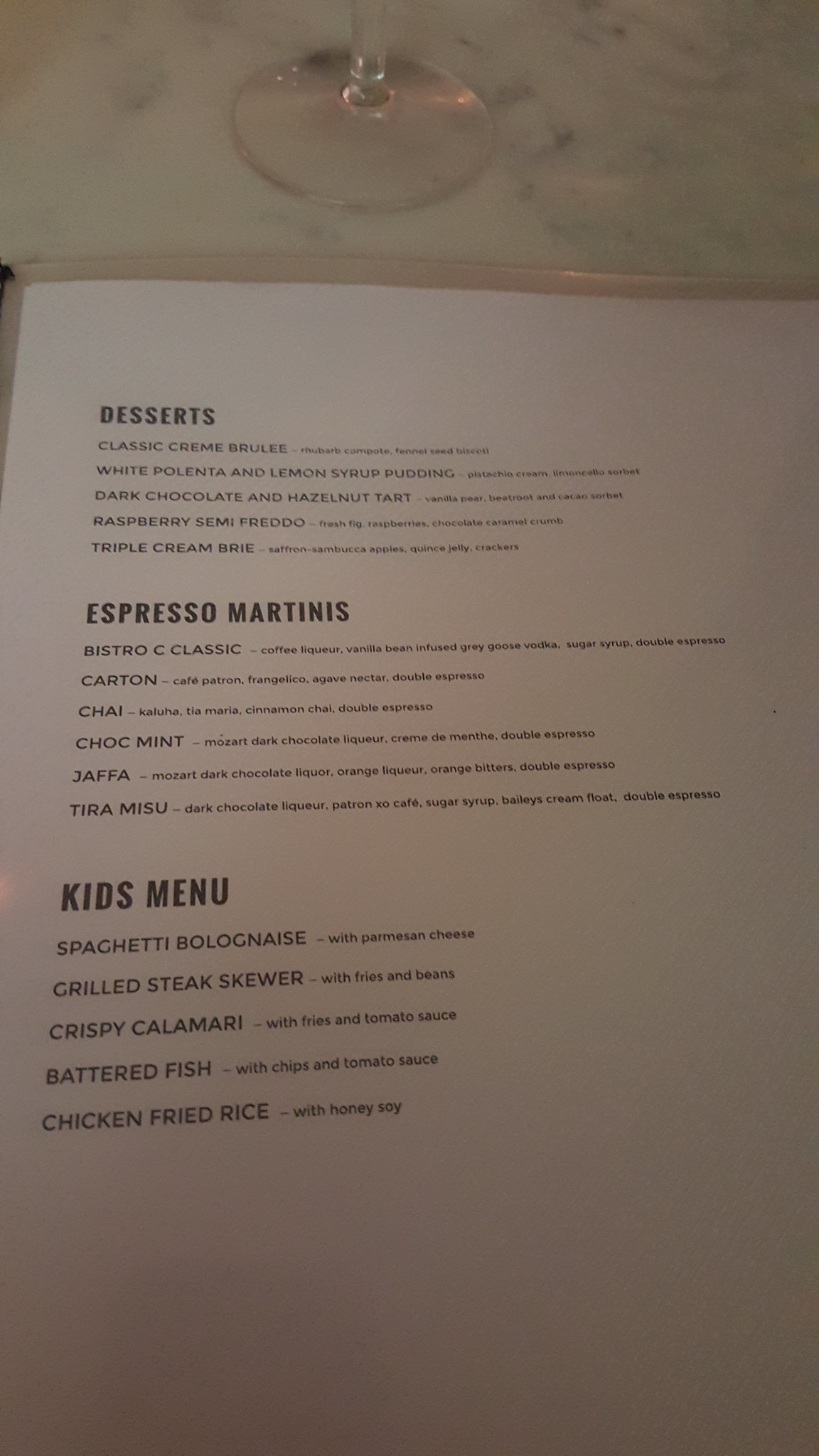An elegant menu rests on a pristine white marble counter, evoking an atmosphere of sophistication, possibly within a bar or restaurant. A wine glass, identifiable by its delicate stem, adds to the scene's refinement, standing partially visible on the counter's surface. The menu, printed on sleek white paper with understated black font, is divided into three distinct sections.

The first section, titled "Desserts," lists an enticing selection including:
1. Classic Crème Brûlée
2. White Polenta and Lemon Syrup Pudding
3. Dark Chocolate and Hazelnut Tart
4. Raspberry Semifreddo
5. Triple Crème Brûlée

Each dessert is accompanied by a tantalizing description, promising an exquisite culinary experience.

The second section features "Espresso Martinis," offering creative variations such as:
1. Bistro C Classic
2. Carton
3. Chai
4. Choc Mint
5. Jaffa
6. Tiramisu

These martinis are detailed with descriptions, hinting at their unique flavors and artistry.

Finally, the "Kids Menu" comprises child-friendly options, each with its own description:
1. Spaghetti Bolognese
2. Grilled Steak Skewer
3. Crispy Calamari
4. Battered Fish
5. Chicken Fried Rice

Overall, the menu exudes simplicity and elegance, with carefully curated dishes and drinks to suit a range of tastes.